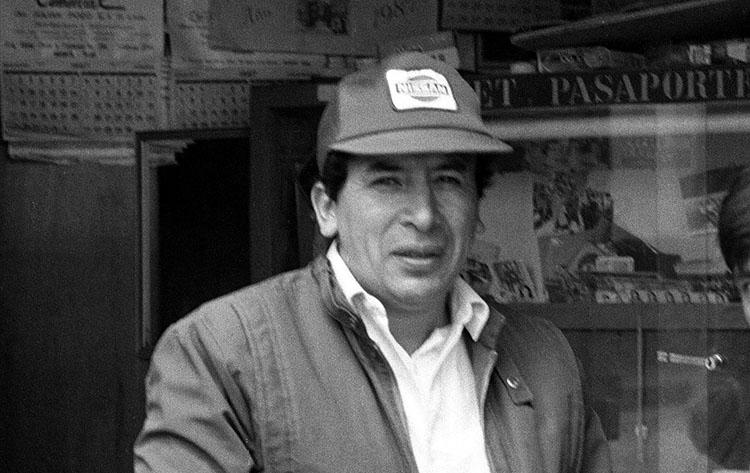This black and white photograph, giving it an old and dated appearance, features a man standing and looking directly at the camera. He has dark hair and thick eyebrows and is wearing a white collared shirt under a jacket. His expression is subtle, with a slight lift to his mouth, which could be interpreted as the start of a smile or squinting. On his head, he wears a baseball cap with an indistinct logo, though it might say "Nissan." The background suggests he is in a cluttered store or some similar setting, with various items and posters, including a sign that reads "PASAPORTE." There are visible objects such as a calendar, a board, and what seems to be glass on the right side. To the right side of the man, another person's partial face, showing an eye and an ear, is visible, although cut off from the frame. The man is in sharp focus, and the lighting highlights him against the detailed but busy background.